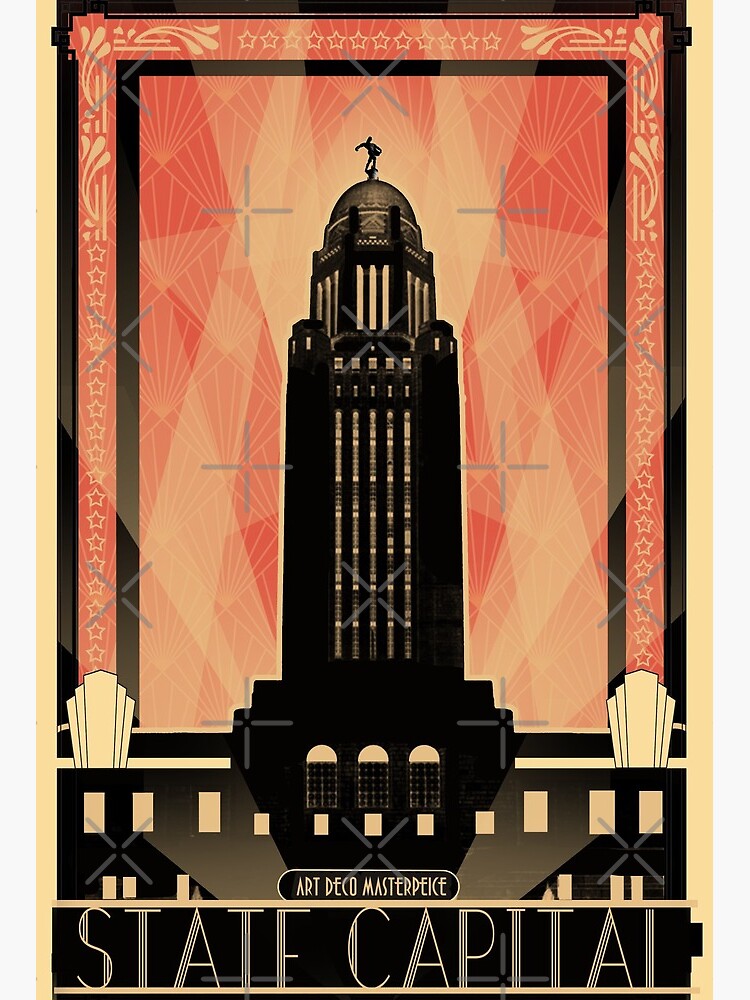The image portrays a meticulously designed Art Deco-style poster, prominently featuring the Nebraska State Capitol building. The focal point of the poster is the stunning depiction of the building, rendered in black and gold hues. The structure is characterized by its towering, columnar form, which culminates in a rounded dome, crowned by a statue of a warrior holding a shield. Vertical windows and imposing pillars accentuate the building's majestic architecture.

The background of the poster is a vibrant gradient of red, yellow, and orange, interspersed with dynamic, angular beams of light and intricate, crisscrossed lines. This colorful backdrop frames the central image, adding depth and intensity. Surrounding the main scene, a border adorned with golden stars, swirled edges, and various Art Deco patterns, including flowers, leaves, and abstract shapes, enhances the vintage aesthetic.

At the bottom of the poster, in a stylized font, the text reads: "Art Deco Masterpiece, State Capitol," highlighting the building's architectural significance. Flanking the central image are two large, fan-like Art Deco motifs, adding balance and symmetry to the overall design. The entire composition is encased within a grey border, providing a refined, elegant outline to this captivating homage to Art Deco artistry.